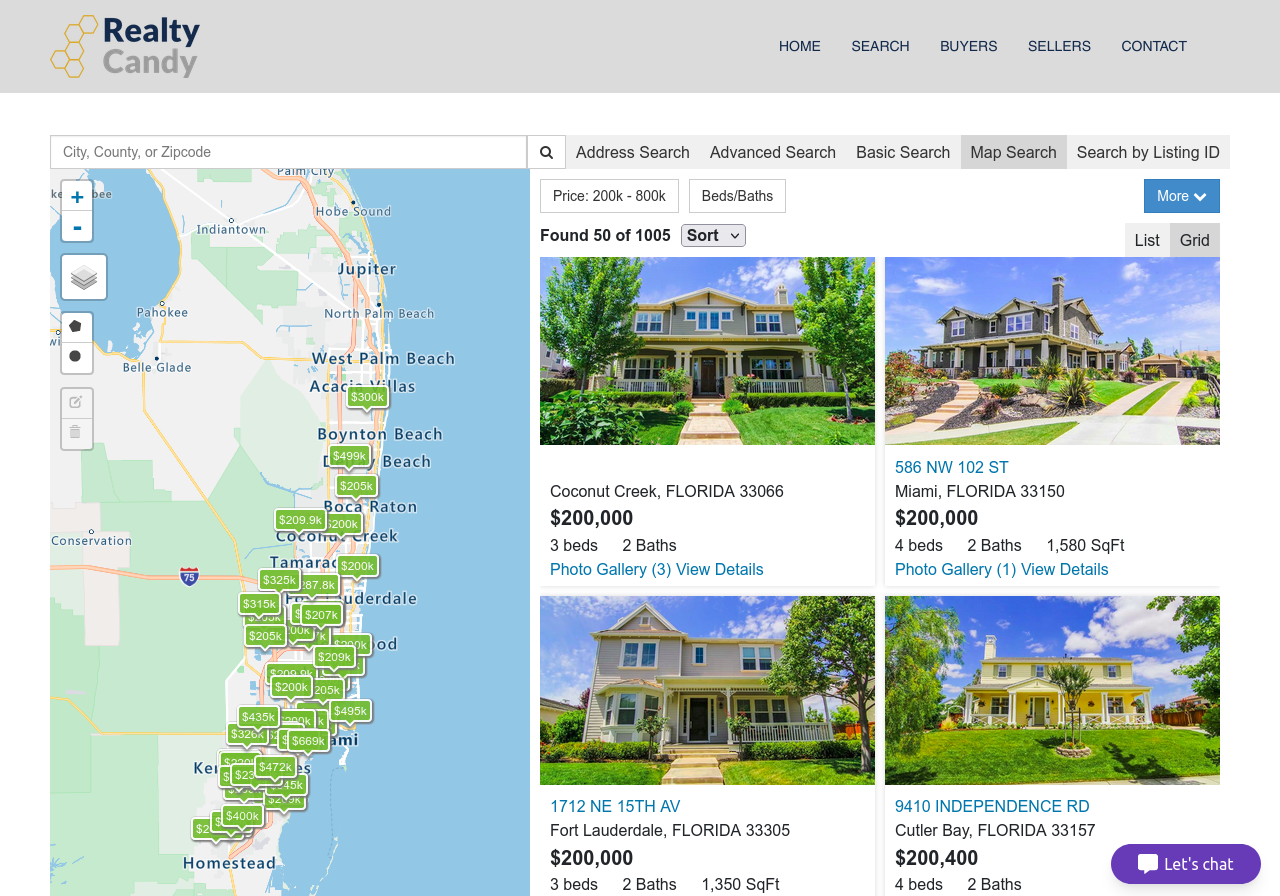Here is a detailed and cleaned-up description for the image:

---

The image, sourced from the website Reality Candy, showcases a listing of real estate properties in Florida with a focus on presenting relevant details for potential buyers. At the very top of the webpage, a gray rectangular header spans across the screen, containing the website's menu options. From left to right, the menu includes links labelled "Home," "Search," "Buyers," "Sellers," and "Contact."

On the left side of the screen, an interactive map of Florida highlights different regions, including a pinpoint for West Palm Beach. Below the map, the website indicates that it has found 50 out of 1,005 available properties.

The main content area features a list of individual property listings. The first listing is for a house in Coconut Creek, Florida, priced at $200,000. The property details reveal it has three bedrooms and two bathrooms, and the listing includes a photo gallery with three images. There is a "View Details" button for more information.

Next, there is a listing for a house in Miami, Florida, also priced at $200,000. This property has four bedrooms and two bathrooms, spans two stories, and includes a photo gallery with one image. The listing specifies that the house measures 1,550 square feet.

Additional property listings continue below, following a similar format, providing users with a comprehensive overview of the available homes.

---